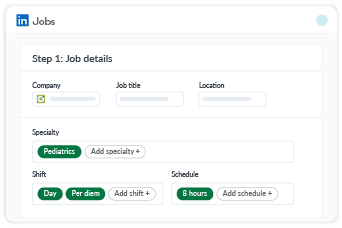The image depicts a form interface for job posting details, encased within a gray-outlined box. In the upper left corner, there's a blue square with the lowercase letters "in" in white, indicating a LinkedIn feature. Beside this blue square, the word "jobs" is written in gray. 

On the far right side of the interface, there is a very light blue circle. Below the "jobs" header, the text "Step One: Job Details" is prominently displayed. Underneath this header, the form begins with the word "company" in black text, followed by an empty green box beneath it. To the right, there are similar fields for "job title" and "location," each accompanied by empty text boxes designed to input respective information.

In the second row, the word "specialty" appears in black text, with an accompanying blue circle containing the word "Pediatrics". Adjacent to this is another circle labeled "add specialty". The final column on this row is labeled "shift," under which there are options displayed as green circles labeled "day" and "per diem". Additionally, there is a white circle displaying "add shift" with a plus sign.

To the right, towards the top of the form, the word "schedule" is shown. Below this, there's a green circle indicating "eight hours" and next to it, a light gray-outlined circle for "add schedule". This detailed layout helps users navigate and fill in job-related information systematically.